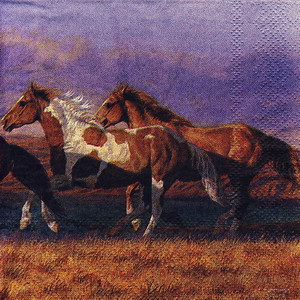In this watercolor or potentially drawn artwork, three horses race dynamically across a field, their tails flapping in the wind. To the extreme left, only the tail and hind leg of a horse are visible, indicating it is exiting the frame. The central horse is a striking light brown with white patches, notably on its mane and face, galloping energetically from right to left. A bit further back and to the right, an all-brown horse with a matching mane and tail follows closely. The foreground features a mix of lush green grass interspersed with yellow wildflowers, while the dark brown and green hues suggest a rugged, potentially evening environment. Rolling hills, or possibly mountains, and a sky awash in shades of purple with puffy clouds, provide a dramatic backdrop, hinting at sunset or early twilight. Trees dot the horizon, completing this vivid portrayal of horses in motion across a natural landscape.